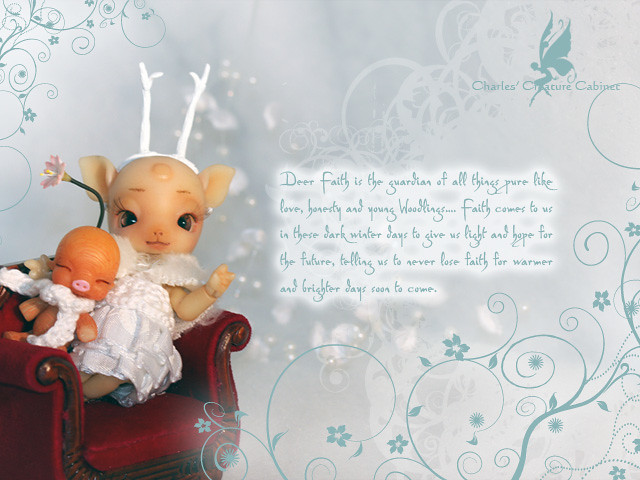The image is a square graphic with a predominantly gray background, subtly blended with light and dark gray tones. It features curlicue vine and floral designs in the upper left and lower right corners, rendered in teal. In the upper right corner, there is text that reads "Charles's Creature Cabinets," accompanied by an illustration of a blue angel or fairy flying over the word "Creature." 

The center of the image contains a poetic message in small, curved teal writing with a glowing white backdrop, making it somewhat challenging to read. The text reads: "Dear Faith is the guardian of all things pure like love, honesty, and young bloodlings. Faith comes to us in these dark winter days to give us light and hope for the future, telling us to never lose faith for warmer and brighter days soon to come."

In the lower left corner, extending up to the middle, there is a red armchair occupied by a small, feminine baby deer-like creature. This creature has white antlers, a plastic-like face with ears, and is dressed in a white outfit. It holds a smaller doll on its lap, which has a pig snout and a flower growing from its head, adding to the whimsical and ethereal atmosphere of the image. The entire composition gives off the impression of a meticulously designed greeting card or a detailed piece of graphic art, conveying themes of hope and purity.